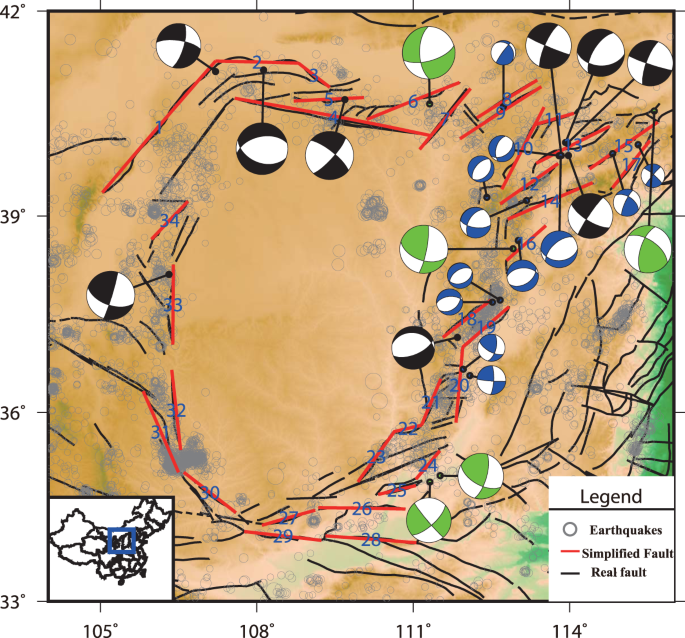This image depicts a square map with a black border and a detailed legend in the bottom right corner identifying different geological features. The map primarily shows a brown landscape with some green areas in the bottom right corner and sporadic blue patches. Scattered across the map are numerous circular symbols resembling beach balls in various colors such as black and white, blue and white, and green and white. These circles represent different earthquakes, with their sizes potentially indicating the earthquake magnitudes. 

The legend clarifies that the circles indicate earthquake locations, a red line signifies simplified faults, and gray lines represent actual faults. Additionally, there are numbers marked along the left side and bottom of the map, ranging from 42 to 114, which help in identifying specific earthquake points. In the bottom left corner of the image, there is a zoomed-out inset map with a blue box highlighting the region depicted in the larger map. This feature offers context by showing the broader geographic location.